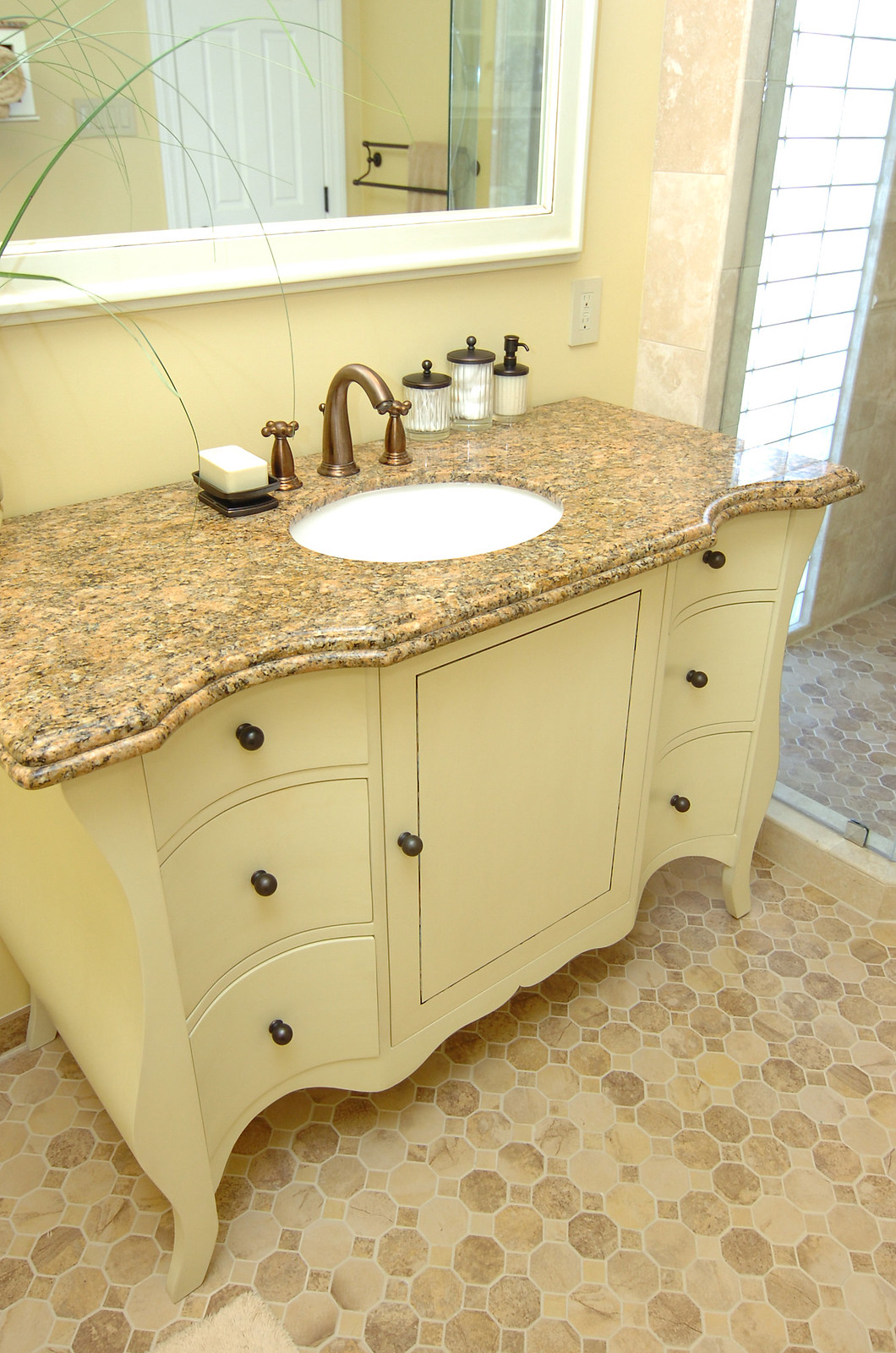The image features a vintage bathroom sink setup atop cabinetry that appears to date back to the late 1940s. The cabinetry is a light yellow color, complemented by black pulls on both the drawers and the door. The countertop is composed of Corian, tinged dark tan with accents of black and darker brown. A burnished brass-colored faucet adorns the sunken white sink.

On the countertop, there are three containers designated for cotton goods: Q-tips, cotton balls, and face pads. A dark brass-colored soap holder with a large bar of soap sits nearby. An electrical outlet is positioned on the wall adjacent to the countertop. Above, a mirror framed in white is mounted on a yellow wall.

The floor is covered in tan vinyl tiles, distinct from the countertop. On the right-hand side of the image, a plant's leaves partially peek into view. A floor-to-ceiling window with obscured subway glass is also visible on this side, adding natural light without compromising privacy.